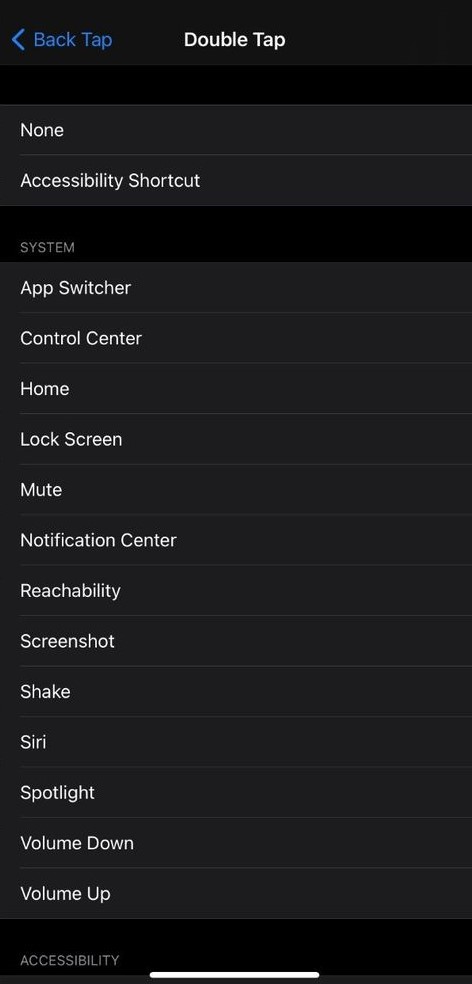The image showcases a predominantly black webpage designed with high contrast and accessibility in mind. At the top left corner, the word "Back Tap" is prominently displayed in blue lettering. Centrally aligned at the top, "Double Tap" is written in crisp white letters. Moving down the page, the first column labeled "None" stands out in white text, followed by "Accessibility Shortcut," also in white. 

Under the "System" section, a series of options are listed in white lettering:
- App Switcher
- Control Center
- Home
- Lock Screen
- Mute
- Notification Center
- Reachability
- Screenshot
- Shake
- Siri
- Spotlight
- Volume Down
- Volume Up

Each option is clearly separated and underlined with a bold white line for emphasis. The entire page uses a subtle gradient of black shades, with the very bottom featuring a darker black background. Here, the word "Accessibility" is displayed in white lettering, accompanied by a long white line extending across the middle bottom part of the page.

The use of varying black tones creates a distinct contrast, allowing the bold white fonts and blue lettering to stand out distinctly, enhancing readability and navigability for users.